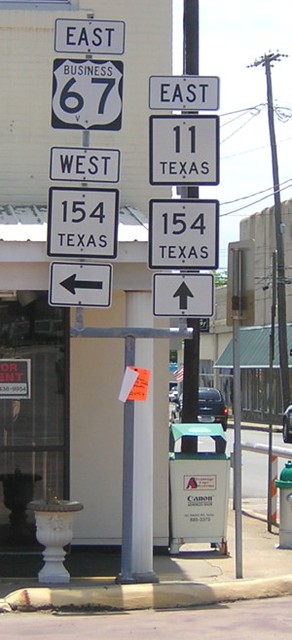The image shows a bustling urban scene with a number of distinct elements. In the foreground to the left, there's a white cement trash bin with black text that reads "Fort Wright" on one side. There's also a white rock with black text underneath. Moving to the right, the street becomes more visible, extending towards a cluster of buildings. One building features a sloped green roof.

An electrical pole with wires stretching horizontally is also visible on the right side. Additionally, there's a pole with several road signs. The top sign indicates directions: the left one says "East," followed by a business route shield reading "Business 67." Below, another sign states "West 154 Texas" along with a left-pointing arrow. Further down, another sign indicates "East 11 Texas" and "5 Texas," with an upward-pointing arrow.

Overall, the scene is rich with urban details, blending infrastructure, signage, and buildings into a lively streetscape.